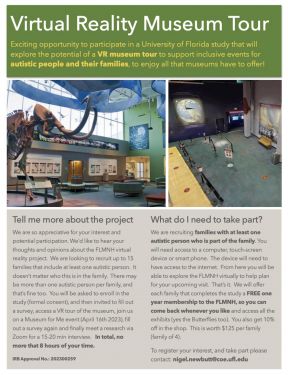This is a detailed flyer for a Virtual Reality Museum Tour, featuring an exciting opportunity to participate in a University of Florida study. The top part of the flyer has a green banner with “Virtual Reality Museum Tour” prominently displayed in bold white text, underlined by yellow text inviting participants to explore the potential of VR tours in supporting inclusive events for autistic individuals and their families. 

Centrally displayed, two photographs showcase the museum's interior: the left photo features a grand exhibit with a reconstructed woolly mammoth skeleton and expansive windows, while the right photo appears to show a more open, possibly under-renovation space. Both images are slightly out-of-focus, contributing to the flyer’s dynamic design.

The body of the flyer is split into two sections. On the left, under the heading “Tell me more about the project” in black text, there is a description outlining the goals and benefits of the study. On the right, titled “What do I need to take part”, the flyer details the requirements for participation, including information about families needing at least one autistic member and the incentive of a free one-year membership to the Florida Museum of Natural History (FLMNH).

In the bottom right corner, contact information is provided for interested participants. The flyer is a vibrant mix of visual and textual information aimed at inviting families to take part in this innovative and inclusive museum experience.